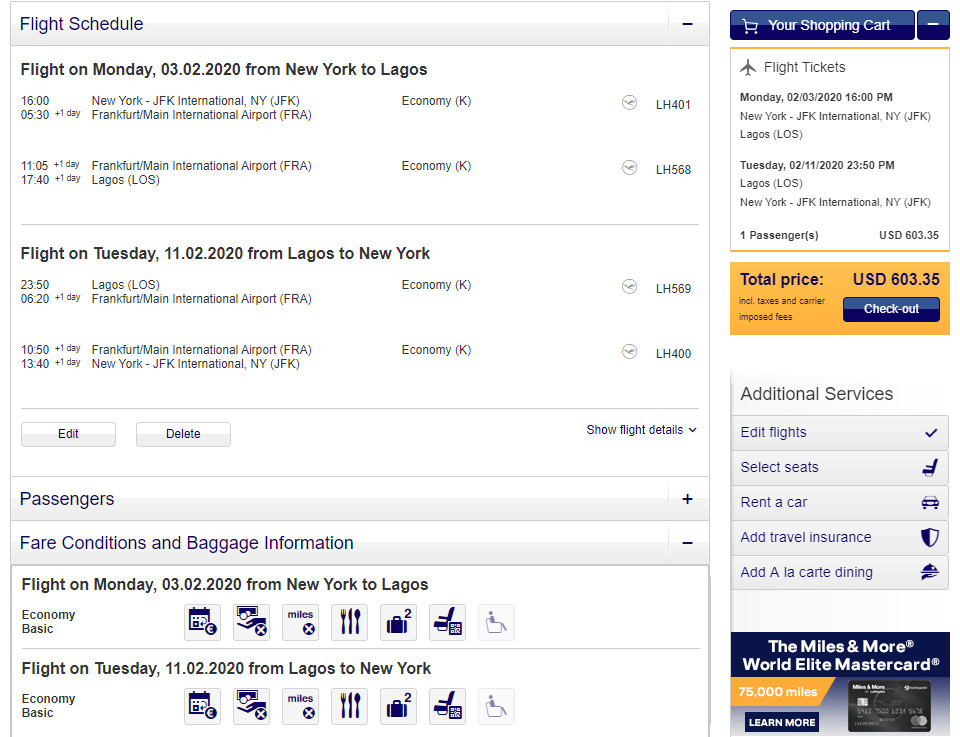**Detailed Description of the Screenshot:**

The screenshot depicts a flight booking interface displayed on a computer screen. In the top left corner, a title reads "Flight Schedule." Directly below this title, a box provides an overview of an outbound flight scheduled for Monday, March 2, 2020, from New York to Lagos. Beneath this outbound flight information, additional flight details are listed.

A second box follows, containing information about the return flight scheduled for Tuesday, November 2, 2020, from Lagos to New York. Below both flight boxes, there are two action buttons labeled "Edit" and "Delete."

On the right-hand side of the screen, there is a dropdown menu labeled "Show Flight Details." Below this dropdown, an expandable "Passengers" section can be revealed or hidden by clicking a plus sign situated to the right. Further down, there is another expandable section labeled "Fare Conditions and Baggage Information," which is fully expanded in the screenshot.

In the top right corner, a section titled "Your Shopping Cart" is visible. This section lists the selected flight tickets and indicates a total price of USD $603.35. A checkout button with a yellow background is prominently displayed beneath the total price.

Underneath the shopping cart section, several clickable links offer additional services. The top link is labeled "Edit Flights," followed by "Select Seats," "Rent a Car," "Add Travel Insurance," and "Add A la Carte Dining." At the very bottom, an advertisement for the "Miles and More World Elite MasterCard" is visible, encouraging viewers to explore this card option.